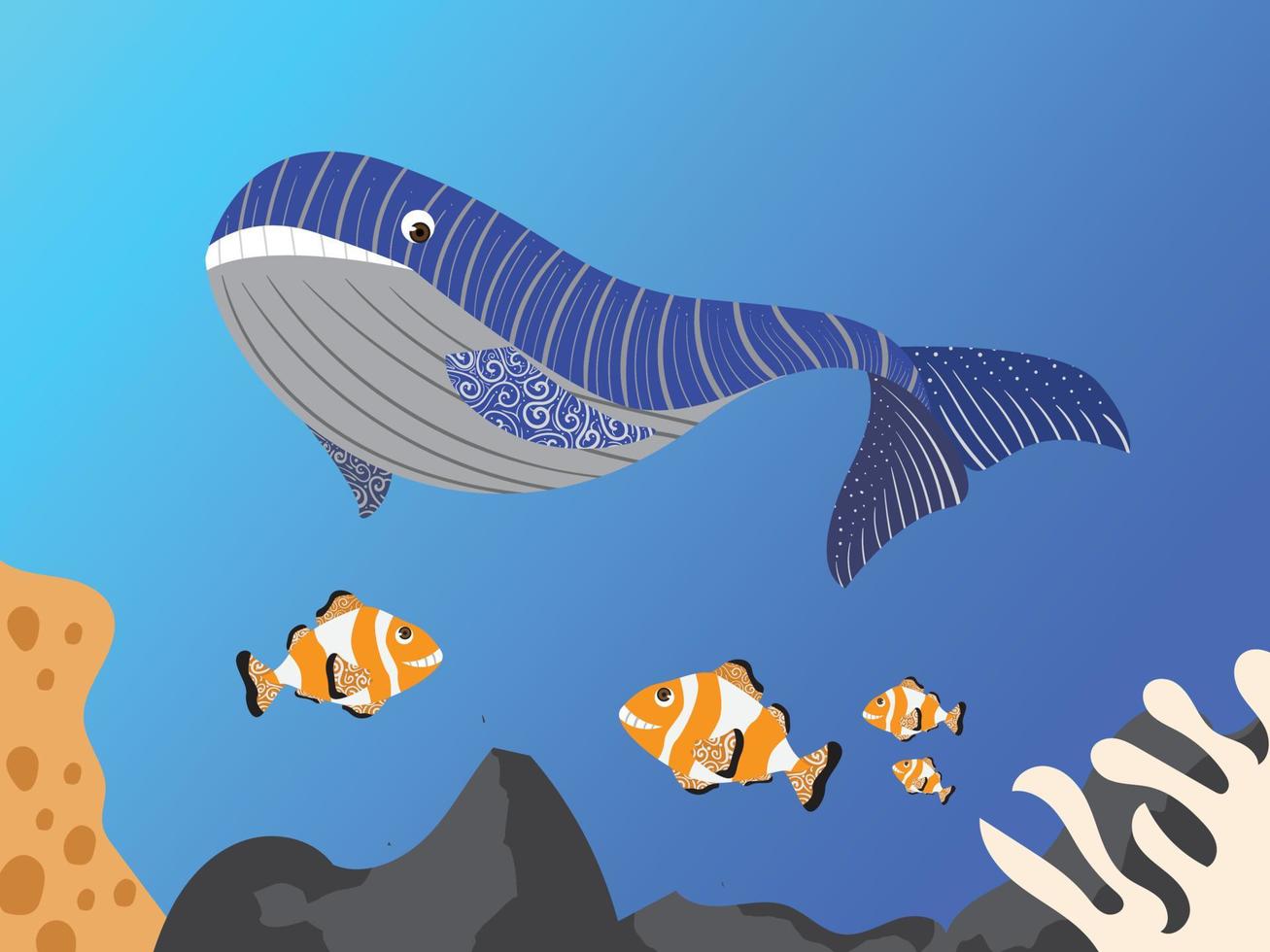This artistic children's book-style drawing depicts an enchanting underwater scene in the deep ocean. The background transitions from a deep blue on the right to a lighter blue on the left. Dominating the upper half of the image is a large, majestic blue whale with a gray underbelly and intricate, swirled white patterns on its fins. The whale's body is accentuated with vertical stripes, in shades of blue and white, giving it a textured appearance. Its dark blue patterned tail and slightly downward smile with white teeth add to its whimsical charm, while its white eye with a black pupil gazes down at the scene below.

Beneath the whale, four orange clownfish, similar in appearance to characters from Finding Nemo, swim joyfully. One fish swims toward the right, while the remaining three swim to the left, all seemingly looking upwards at the whale with cheerful expressions.

At the bottom of the image, the ocean floor is adorned with black and gray rocks. The bottom left corner features a light orange, porous coral structure, and on the bottom right, a pristine white coral stands out against the darker rocks. The detailed and vibrant elements of this scene bring the underwater world to life, capturing the imagination and wonder of an undersea adventure.